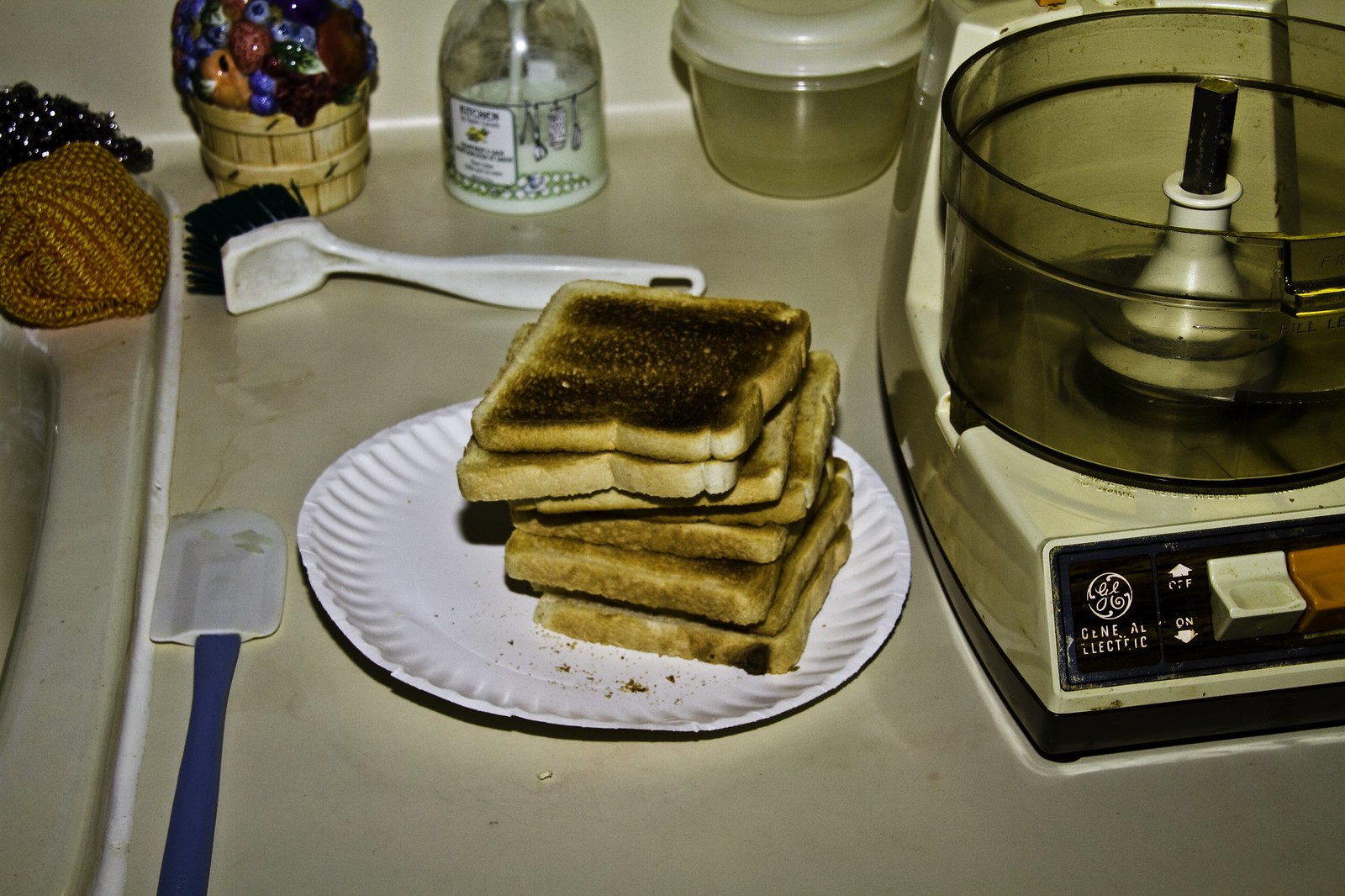The image, likely from a kitchen that hasn't been renovated since the 1970s or possibly an actual snapshot from the era, features a cluttered countertop adjacent to the sink. Centered on the counter is a white paper plate holding a stack of eight toasted slices of bread, with the top piece noticeably more browned in the center. To the left of the plate lies a flat spatula with a blue handle and white rubber blade. Beside the toast is a General Electric electronic appliance resembling an old-fashioned food processor or popcorn popper, characterized by an on/off switch with white and orange buttons and a central stirring or popping mechanism, but missing the mixing attachment. In the background, various items contribute to the retro kitchen tableau: a long brush with black bristles for cleaning dishes, a Tupperware container possibly filled with water, and a bottle that appears to contain soap or lotion. There is also a decorative glass fruit basket adding a nostalgic touch to the scene.